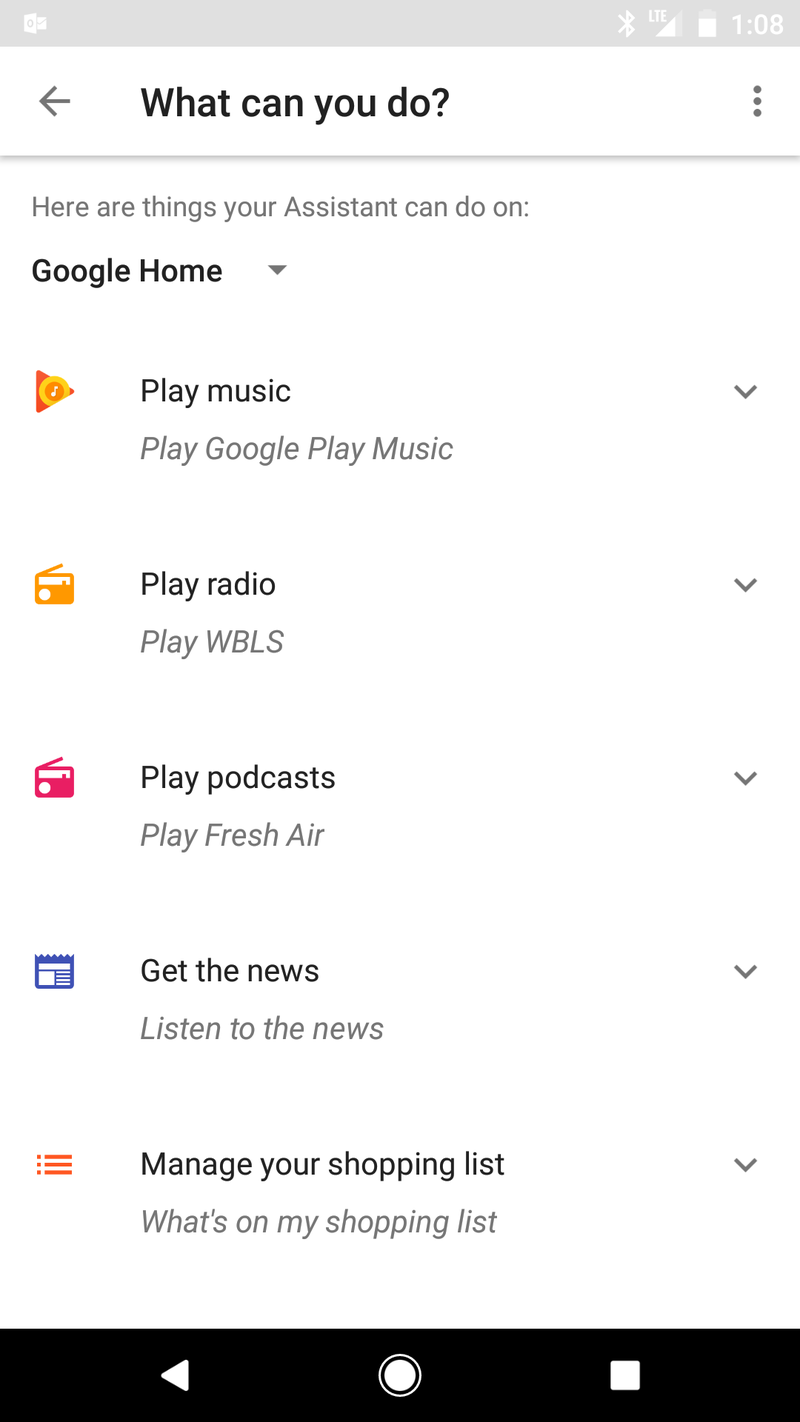This image is a mobile screenshot with a predominant white background. At the bottom, there is a solid black banner, and at the top, a very light gray thinner banner. The top left corner features an icon, while the top right corner displays multiple icons including a Bluetooth symbol, LTE connection indicator, battery level icon, and the time showing 1:08.

Directly beneath, a bold black header reads "What can you do?" with a left-pointing arrow adjacent to it. Following this header, there is text that reads, "Here are some things your assistant can do on," with "Google Home" underneath, accompanied by a downward arrow.

The main content area features five colorful icons in blue, pink, and orange, associated with a list of actions. These actions include playing various types of audio content such as music ("Play music," "Play Google Play Music," "Play radio," "Play WBLS," "Play podcasts," "Play fresh air"), accessing news ("Get the news," "Listen to the news"), and managing a shopping list ("What's on my shopping list").

Adjacent to these sections are scroll bars indicating additional information can be viewed by scrolling. The bottom black banner houses three navigational buttons: a white filled-in left arrow, a white filled-in circle, and a white filled-in square.